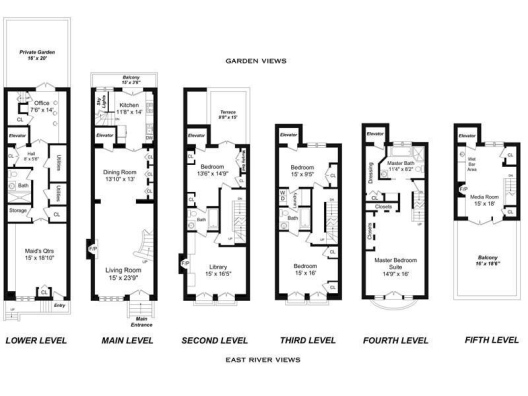An elaborate floor plan of what appears to be a luxurious five-story apartment complex titled "East River Views" is depicted in this image. The lower level includes a detailed floor plan with a private garden, maid's quarters, and other defined rooms outlined in bold black lines. The main level features a spacious living room, a well-equipped kitchen, a formal dining room, and an inviting balcony. The second level showcases a terrace, a cozy bedroom, a well-stocked library, and room dimensions clearly labeled. Moving to the third level, there are two bedrooms and a bathroom, alongside a small balcony. The fourth level is dedicated entirely to the master suite, comprising a master bedroom, a lavish master bath, and an elevator access point, which is noted to be available on all floors. The fifth and final level boasts an expansive balcony that occupies a significant portion of the floor, with indicated options for customizable features.